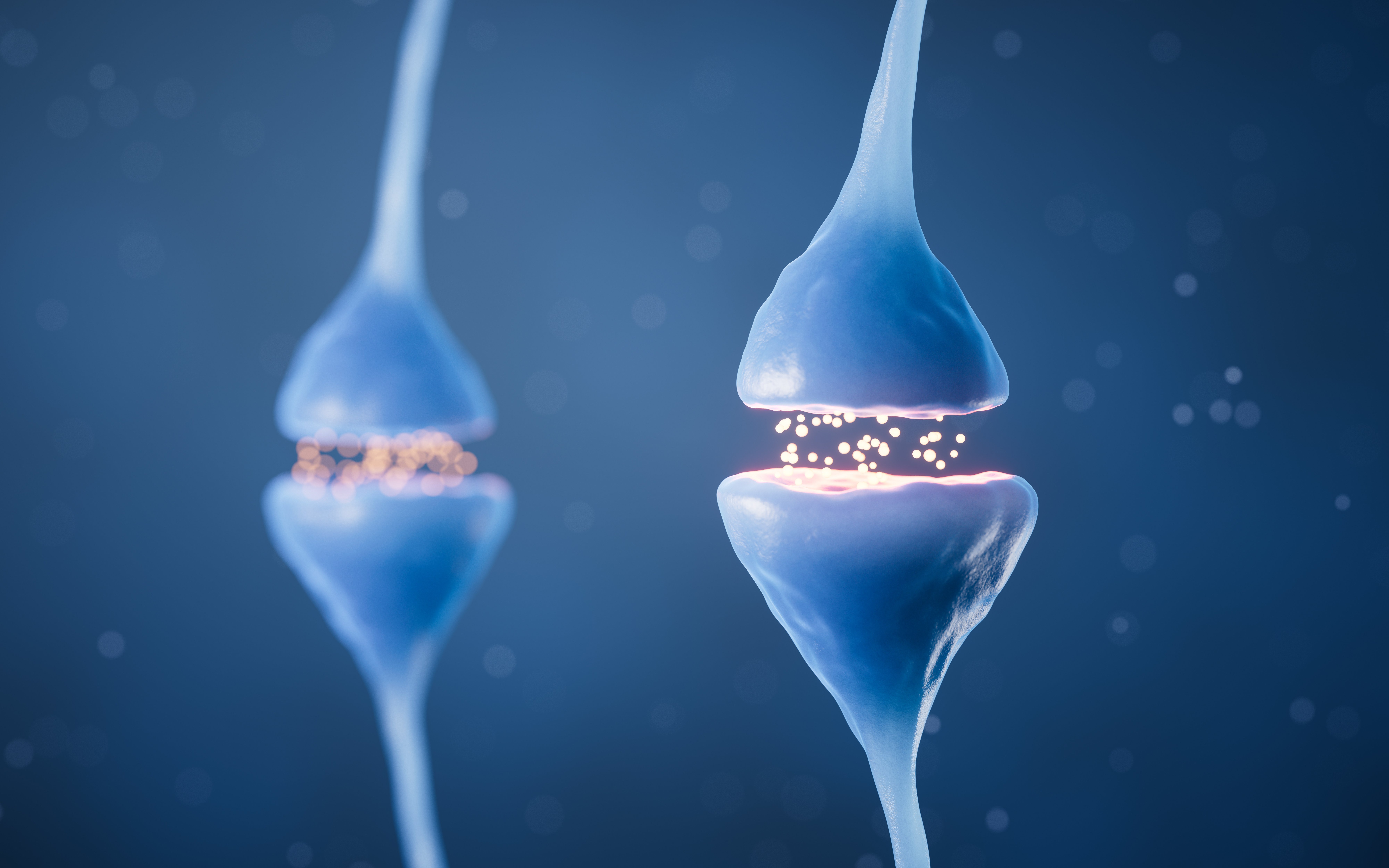This digital illustration depicts a vivid blue, three-dimensional scene that resembles synaptic connections within the brain. The visual centers on two funnel-shaped structures, reminiscent of neural synapses, with the one on the right in sharp focus and the other on the left slightly blurred to suggest depth. Both synapses are depicted in a striking bright blue color with delicate material textures, contrasting against a dark blue background. Between these structures, various particles float—some appearing as little white dots while others are orange or pinkish—that suggest electrochemical energy being exchanged. The right synapse features more distinct white particles, whereas the left synapse shows larger, beige or lighter-colored dots. The overall effect is visually striking, creating an eye-catching, immersive depiction of synaptic activity in the brain.